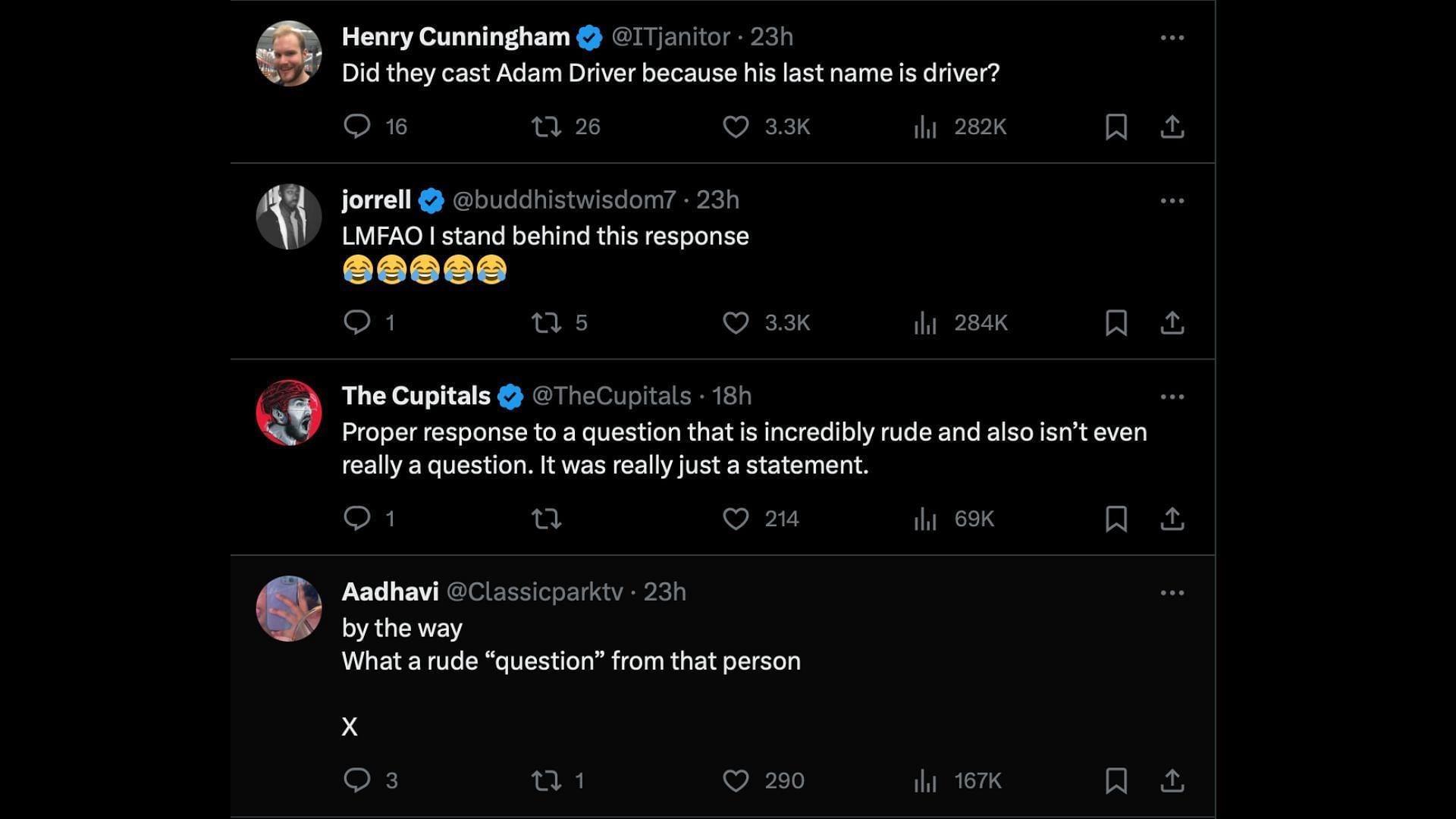In a lively social media exchange, Henry Cunningham, verified IT janitor, humorously inquired, "Did they cast Adam Driver because his last name is Driver?" This light-hearted comment garnered significant attention with 16 comments, 26 shares, and 3,000 likes. Choral, under the handle BuddhistWisdom7, responded with amusement, saying, "LMFAO, I stand behind this response," accompanied by five laughing-crying emojis, earning one comment, five shares, and matching the 3,000 likes of the original post.

Another verified user, TheCupitals, weighed in, describing Henry's remark as a "proper response to a question that is incredibly rude and also isn't even really a question. It was really just a statement." Adhavi from Classic Park TV echoed this sentiment, quoting, "By the way, what a rude question," and receiving three comments and 290 likes for their contribution to the dialogue.